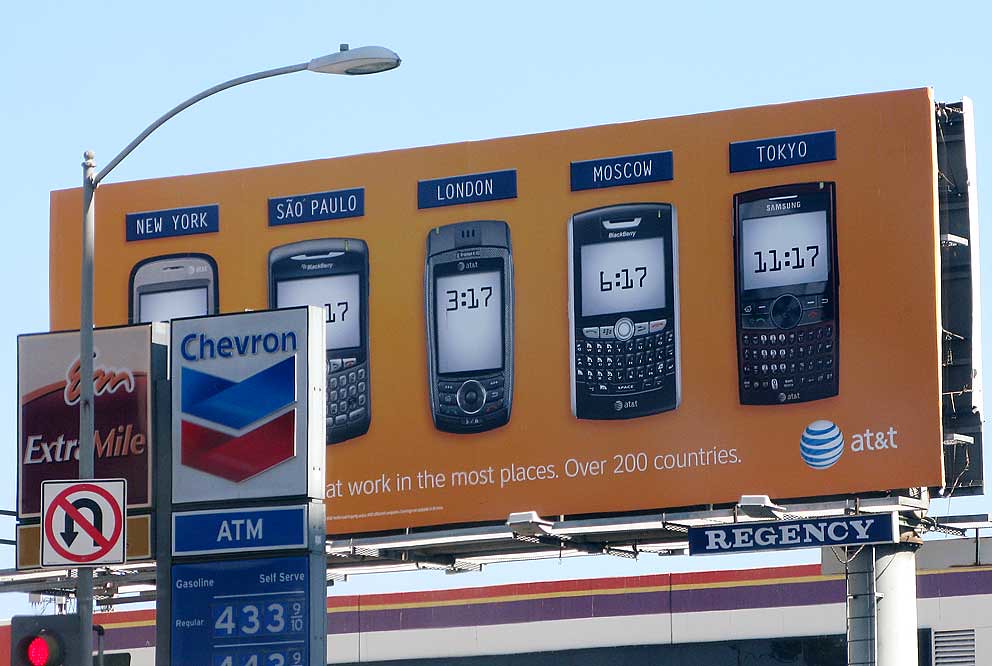In the foreground of this vibrant photograph stands a large Chevron gas station sign, proudly displaying the price of regular gas at $4.33 and nine-tenths. A street light adjacent to the sign features a no U-turn sign and a red light. The scene is set with the partial view of an urban building in the background.

The main focus of the image is a striking orange billboard advertising AT&T services. The billboard showcases five distinct cell phones, likely including brands like BlackBerry, Nokia, Samsung, and perhaps Nextel, each stationed to represent different international cities: New York, Sao Paulo, London, Moscow, and Tokyo. The times displayed on the phones are 3:17 for London, 6:17 for Moscow, and 11:17 for Tokyo, while the times for New York and Sao Paulo are obscured by the Chevron sign.

At the bottom of the billboard, partially covered but visible, the text reads, "Work in the most places. Over 200 countries." This is followed by the recognizable AT&T logo and the word "Regency." The juxtaposition of global connectivity provided by AT&T with the local, familiar sight of the gas station creates an intriguing blend of local and international elements, suggesting seamless communication no matter where in the world one goes.